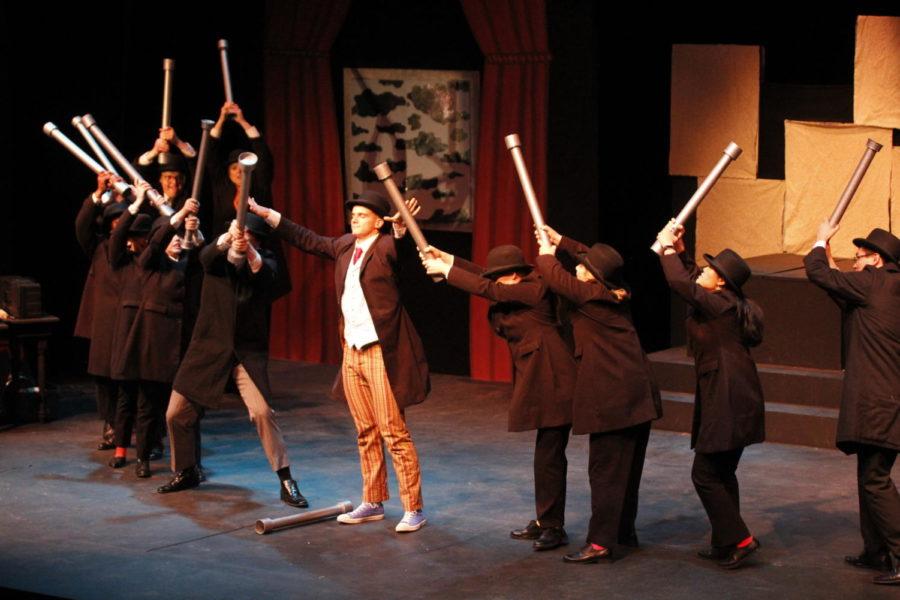The image captures a dramatic scene from a theater play, focused on the central character—a man wearing a three-quarter length brown coat, a white shirt, a red tie, and orange-striped pants paired with tennis shoes. He strikes a pose with his arms raised out to the sides and appears to have his eyes closed. This man, possibly wearing a black hat, stands on a dark-colored stage floor. Surrounding him are several individuals, including what may be children or smaller people, all clad in dark-colored coats and hats—possibly bowler hats—and dark slacks. Each of these individuals holds a metal pipe-like tool aloft, seemingly poised to strike, while the main character's own tool lies discarded on the floor. Behind this tense tableau, red curtains frame a backdrop depicting clouds, with black steps of a staircase visible at the right edge of the stage, adding depth to the theatrical setting. The scene is richly detailed, illustrating a pivotal moment in the narrative of the play.